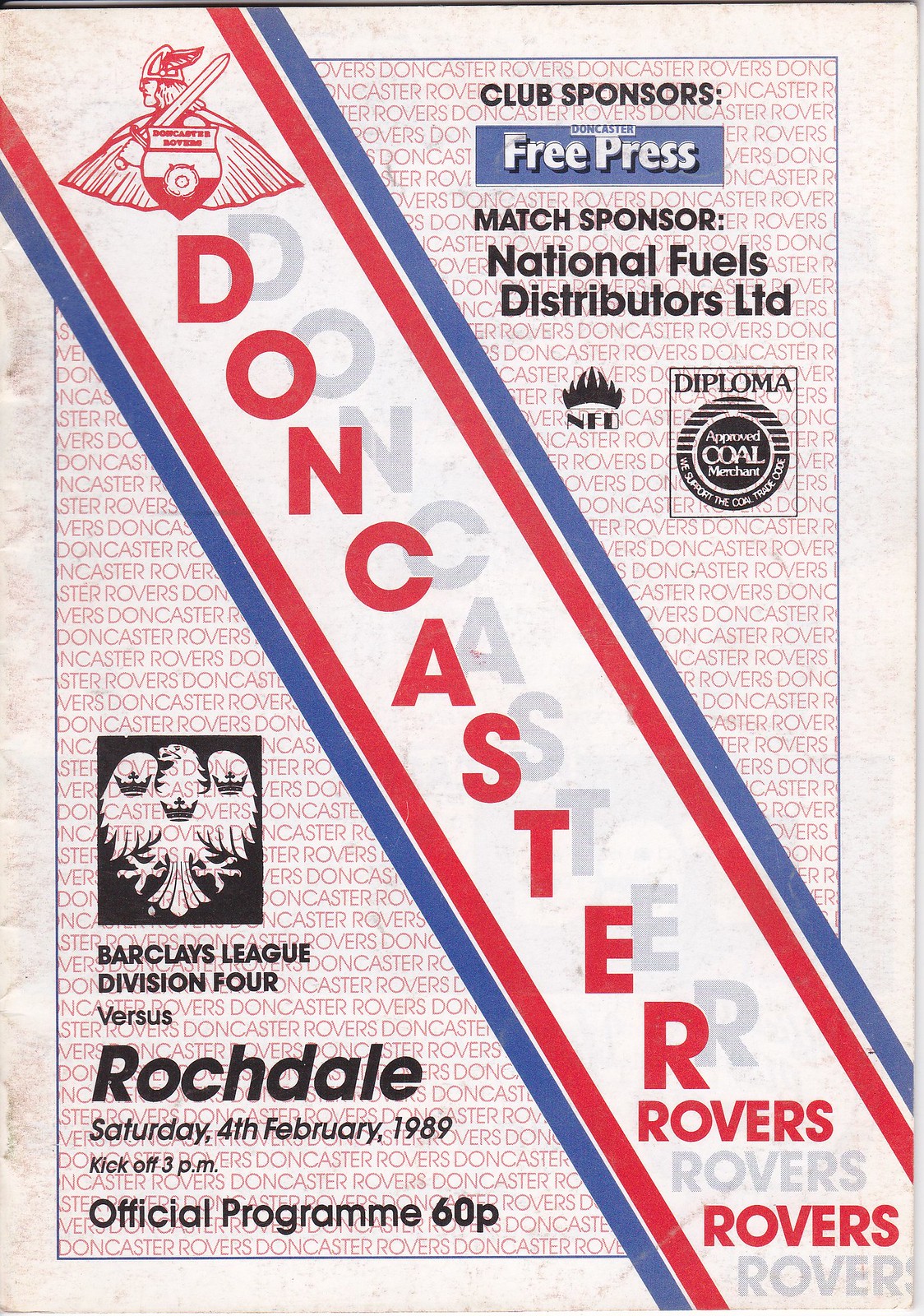This image features a poster, prominently displaying the text "Doncaster Rovers" in bold red lettering, running diagonally from the top left to the bottom right. The red text is shadowed by gray, creating a striking effect against the white background. The poster has red and blue stripes bordering each side. The entire background is overlaid with a repeated light red "Doncaster Rovers" text pattern. 

At the top right, the text "Club Sponsors" is displayed in black, followed by a "Free Press" logo on a blue background. Below this, "Match Sponsor: National Fuels Distributors, LTD" is printed in black. Additionally, on the bottom left, there is a black-outlined logo featuring a bird with crowns, signifying the Barclays League Division 4. Important match information is noted: “vs. Rochdale, Saturday 4th, February 1989, kick-off at 3 p.m., Official Program 60 pence.”

An outlined Viking image is also situated on the top right, enhancing the heritage aesthetic of the poster. This is the official program cover for the Doncaster Rovers' soccer match, meticulously detailing sponsors and game specifics.